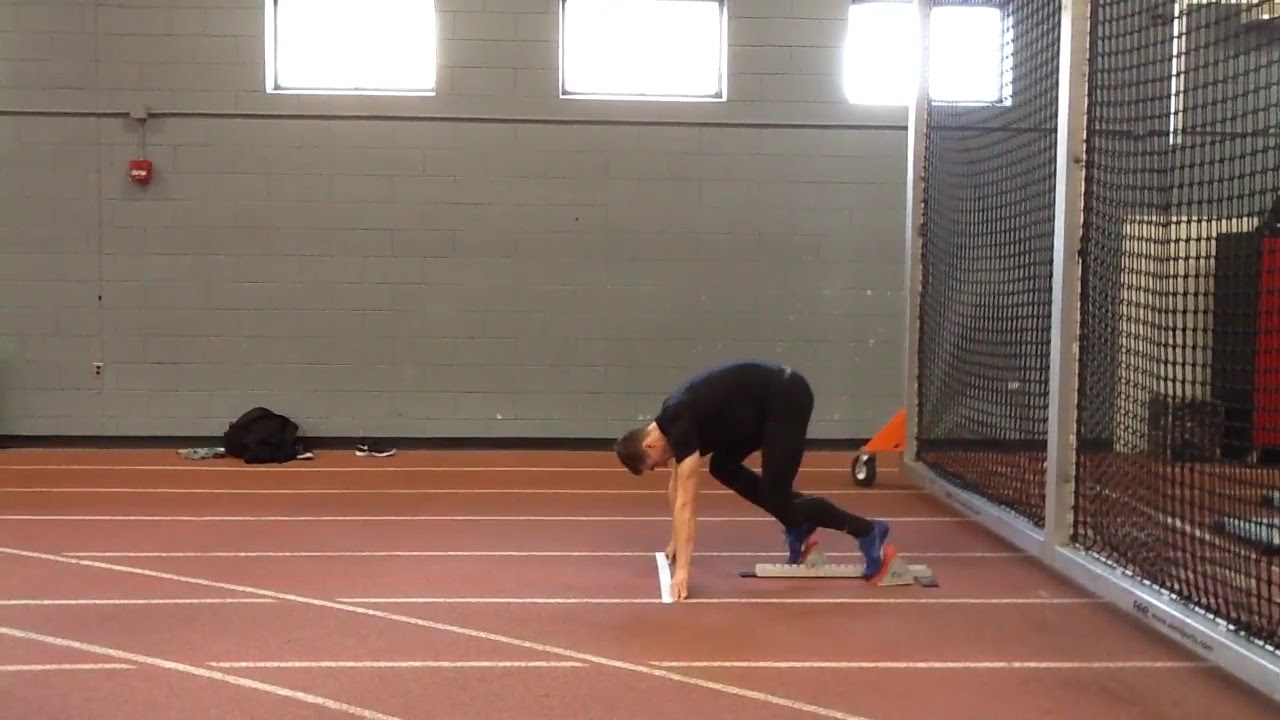This photograph depicts an indoor running track that runs horizontally across the image. The track is maroon in color with white lines marking seven lanes. Positioned in the third lane, a man in a black shirt and black pants is preparing to sprint, adopting the classic runner's stance with his hands on a white line and his feet on a starting block. He has blue shoes, medium dark hair, and his head is completely down, focused on the start.

Behind him, the wall of the gymnasium is white with a pattern of rectangular bricks, featuring three large windows at the top through which bright sunlight streams, casting a glare on the scene. To the left of the man, there's a red fire alarm box and an outlet on the pavement gray wall, and some belongings including a black bag and a pair of black tennis shoes are scattered on the floor. On the right side of the image, a net structure, framed by a metallic framework with wheels, suggests it can be moved or adjusted as needed.